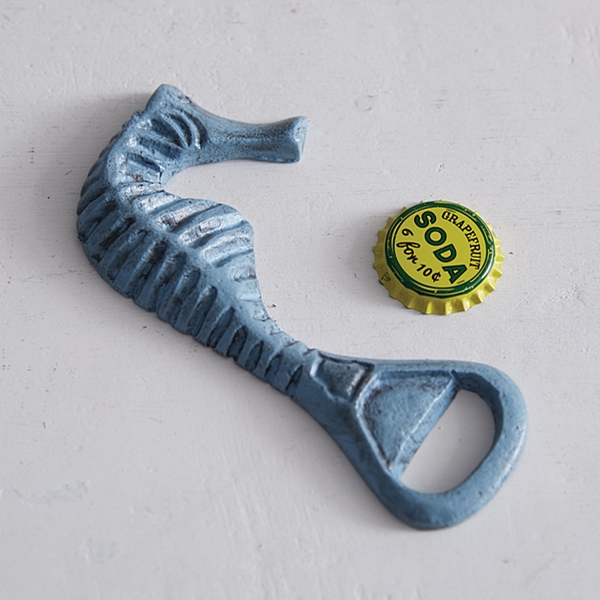The photograph features an antique bottle cap opener crafted in the shape of a seahorse, lying on an off-white surface. The opener, painted in a light denim blue color, appears to be made of sturdy ceramic or stone with horizontal ridges along the seahorse's body. The seahorse's head is positioned in the upper left corner of the image, curving gracefully down towards the lower right where its curled tail forms the functional part of the tool. This crudely detailed, yet charming seahorse boasts a long, narrow snout. To the right of the bottle opener lies a round, yellow metal bottle cap with a green ring around the center. The cap reads "grapefruit" in black letters at the top, "soda" in green letters beneath it, and "six for ten cents" in black letters at the bottom, encircled by yellow ridges. The overall layout of the photograph is nearly square.